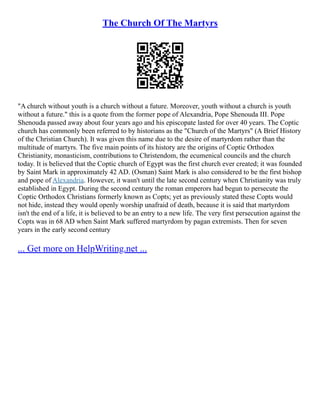The image features a QR code prominently displayed beneath the title "The Church of the Martyrs." Accompanying the QR code is a descriptive paragraph containing a quote from the former Pope of Alexandria, Pope Shenouda III: "A church without youth is a church without a future. Moreover, youth without a church is youth without a future." This meaningful quote reflects Pope Shenouda III's deep connection to the church, where he served for over 40 years until his passing approximately four years ago. Additionally, the text mentions the historical context of the Coptic Church, often referred to as the Church of Martyrs, highlighting key dates such as 42 AD and 68 AD associated with Saint Mark and Alexandria. For further information, readers are directed to visit the link provided at the bottom of the paragraph: getmoreonhelpwriting.net.